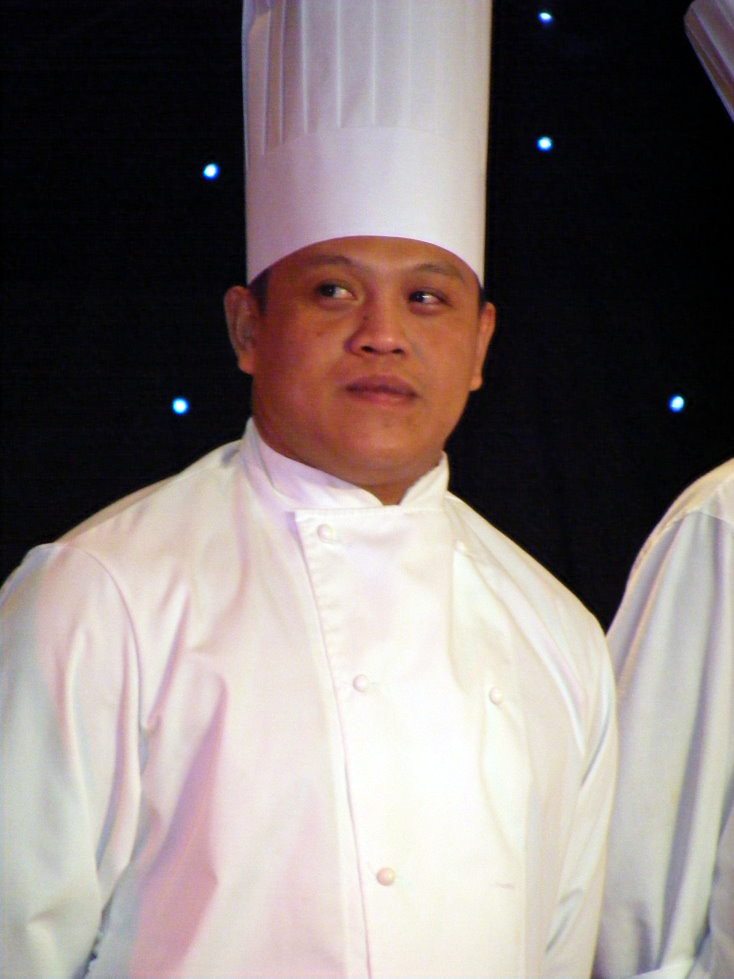In this close-up portrait photograph, a young, clean-shaven chef of Asian descent stands in the foreground, his figure captured from the waist up. He wears a pristine white chef's jacket adorned with a collar and three visible white buttons, along with a tall, white chef's hat that appears to be at least a foot high. The chef has dark skin, black hair, and brown eyes, and his lips are closed in a slightly amused expression. He gazes off to his right, which corresponds to the left from the viewer's perspective. Beside him, we see the left arm and shoulder of another chef, also clad in a white chef's jacket. The background features a black curtain with several small white lights that resemble stars scattered behind and around the chef's hat and shoulders, adding a subtle, almost ethereal touch to the scene.